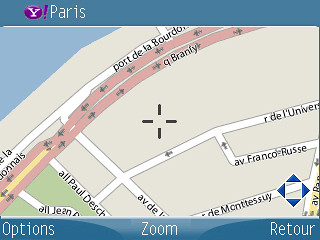This image is an old screenshot from a Yahoo mapping service, likely a GPS system on a computer. The interface features a blue bar at the top and bottom. The top bar displays the Yahoo logo, consisting of a white capital "Y" with a purple background and a purple exclamation point next to it. Beside the logo, "Paris" is written in white letters. The bottom bar includes three options in white font: "Options" on the left, "Zoom" in the middle, and "Retour" on the right. In the bottom right corner, there are four blue directional arrows pointing up, down, left, and right.

The map itself, centered on an overhead view of Paris streets, includes multiple named roads in French. A crosshair marking the center of the map contains intersecting black lines extending in four directions. Notable features include a pinkish main road with directional arrows and green areas likely representing parks. A red line with arrows suggests a specific route, possibly along the River Seine, indicated by a curved line with adjacent blue areas. One visible street name is "Avenue Franco Rousse."